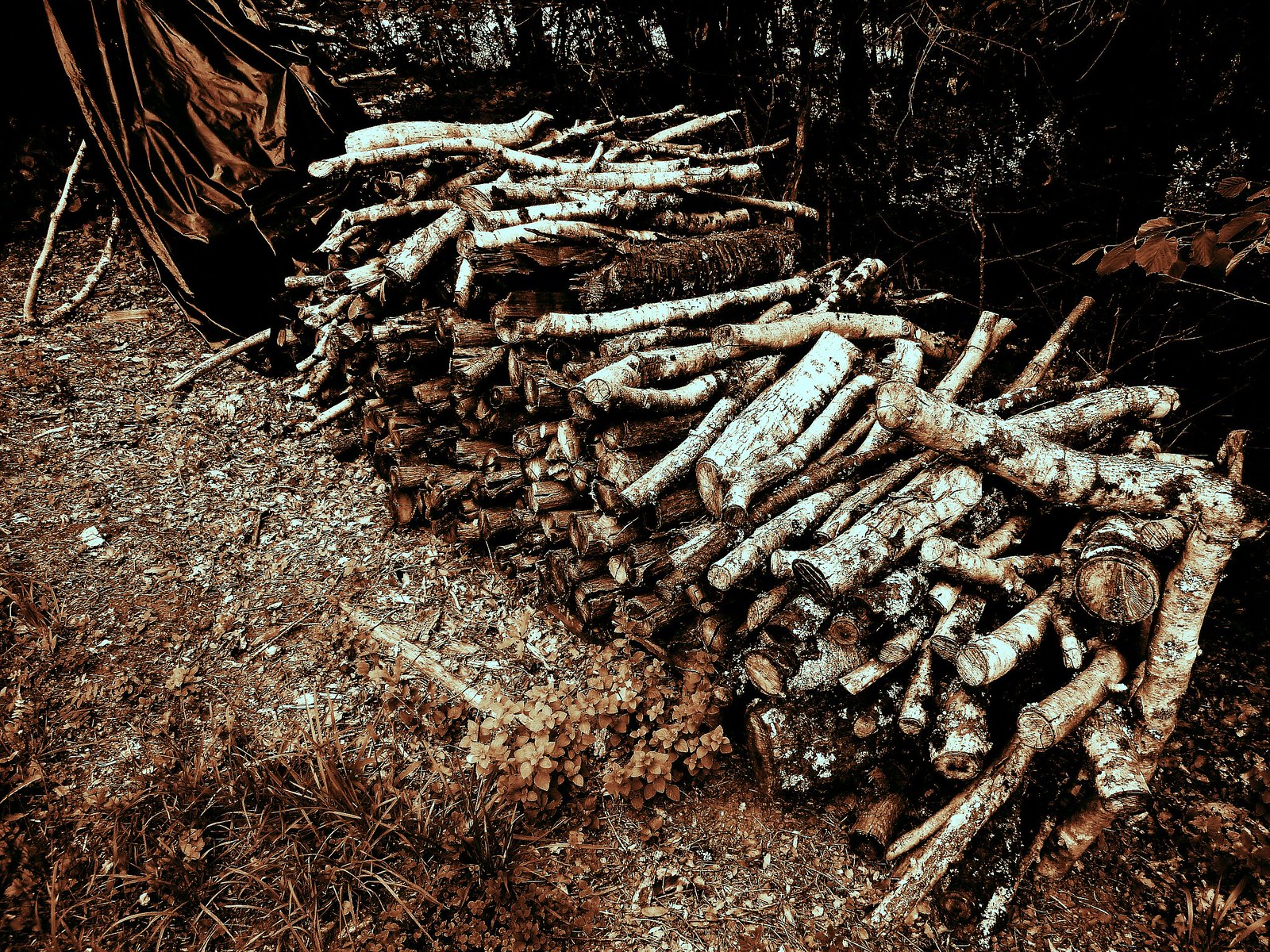In this outdoor photograph, the setting is a serene woodland area during what appears to be autumn. The focal point is a neatly stacked, rectangular pile of logs, all cut to similar lengths, suggesting they are prepared for firewood. The logs, predominantly white in color with hints of birch bark, are piled in a somewhat box-like shape. The ends of the logs exhibit clean, straight cuts, indicative of saw use. The ground beneath the pile is strewn with brown leaves and wood shavings, adding texture to the autumnal scene. In the lower left foreground, a set of bushes adds a touch of greenery, contrasting with the brown and white tones of the logs. The background features a dense forest with dark tree trunks, through which only a sliver of light filters, enhancing the photograph's tranquil and rustic atmosphere. No text or people are present in the image.